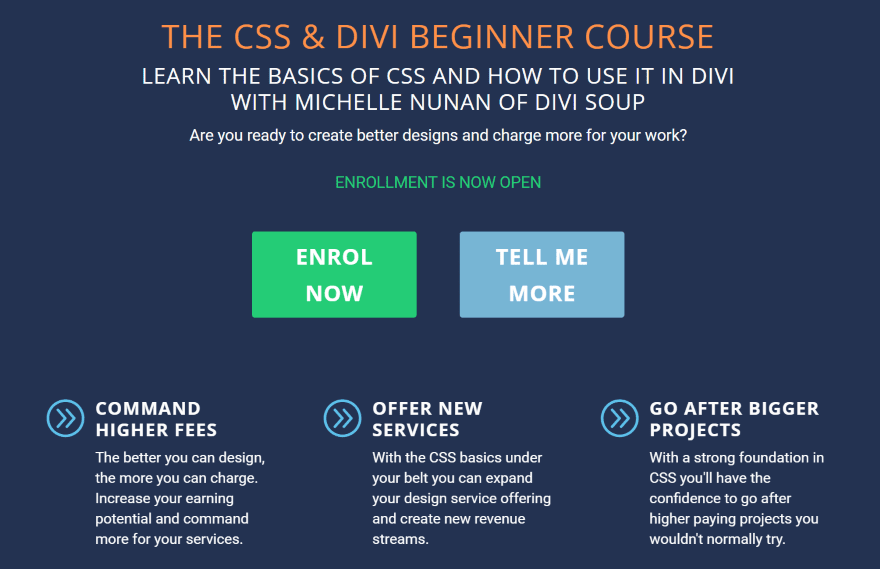The image is a large, visually appealing advertisement for a beginner course in CSS and DEIBI, styled to cover the entire webpage. The main title, written in bold orange text, reads, "CSS and DEIBI Beginner Course." This title is prominently displayed inside a substantial blue box, making it eye-catching.

Below the main title, a white text block provides additional details: "Learn the basics of CSS and how to use it in DEIBI with Michelle Nunn, DEIBI Suit. Are you ready to create better designs and charge more for your work?"

Following this, green text announces, "Enrollment is now open." Immediately below this announcement are two actionable buttons: a green box with "Enroll Now" written in white text, and a pewter blue box with "Tell Me More" also in white.

At the very bottom of the image, three key benefits are listed to entice potential students: 
1. "Command Higher Fees" 
2. "Offer New Services" 
3. "Go After Bigger Projects"

Each of these benefits is accompanied by a double right arrow encircled in light blue, providing a cohesive design element that guides the viewer's eye and emphasizes the points made.